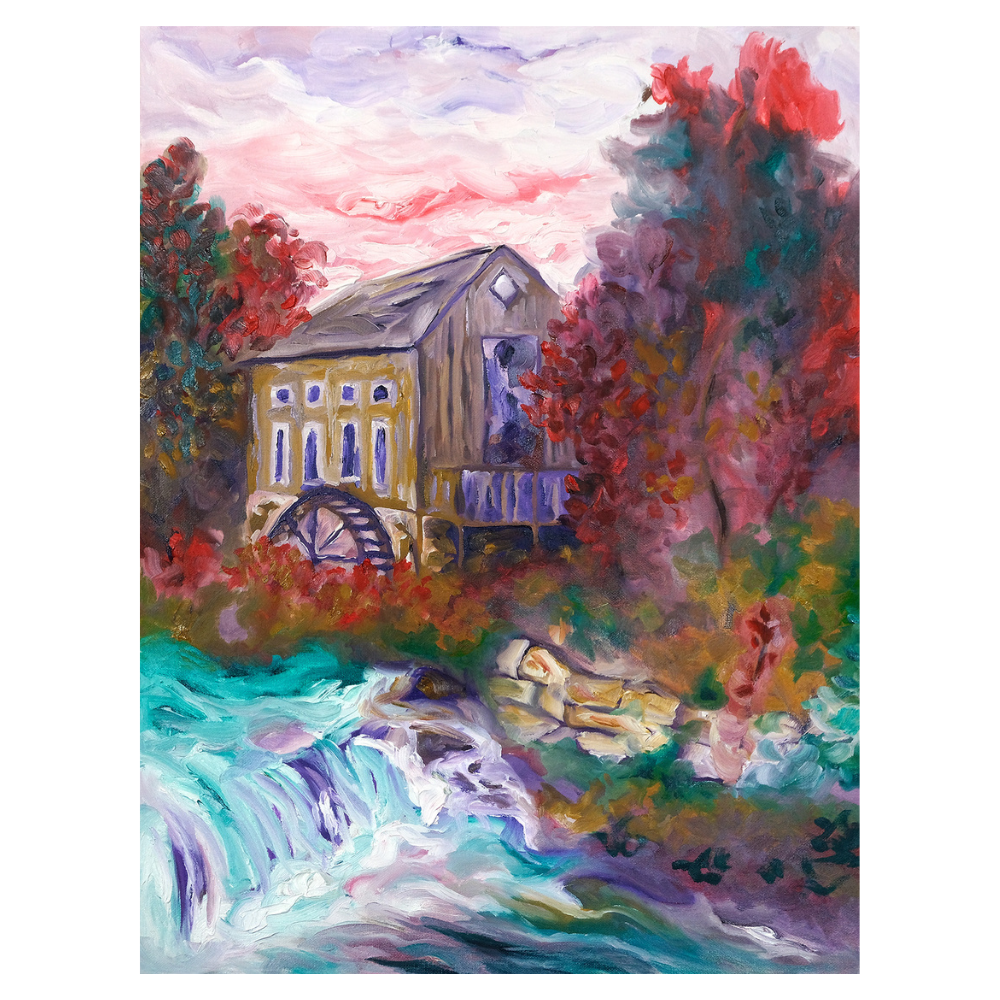This is an impressionistic watercolor painting of a picturesque gristmill, nestled within a vibrant and colorful landscape. The sky at the top of the painting is an ethereal blend of lavender, pink, white, and touches of red, descending towards the horizon where it meets the structure. The gristmill itself is a relatively small, house-like building with a gray-white roof and mustard yellow walls adorned with blue windows. A distinctive water wheel is attached to the side of the gristmill, hinting at its utility.

Tall, slightly abstract trees flank the mill on both sides. The trees on the left are darker and greener with bursts of red, while the trees on the right predominantly showcase red leaves interspersed with patches of light blue and green. Some trees even extend significantly into the sky, with multicolored leaves varying from deep reds and yellows to greens and blues.

In front of the gristmill flows a dynamic river, depicted with an array of aqua, turquoise, light and dark purples, and teal blue tones, creating a vibrant contrast with the warmer hues of the surrounding foliage. Accented with pavers along its edge and a hint of a rushing waterfall, the river adds a sense of movement and liveliness to the scene. Red flowers and a reddish-yellow grass-like area add further splashes of color in the foreground, enhancing the overall vibrancy and charm of the painting.